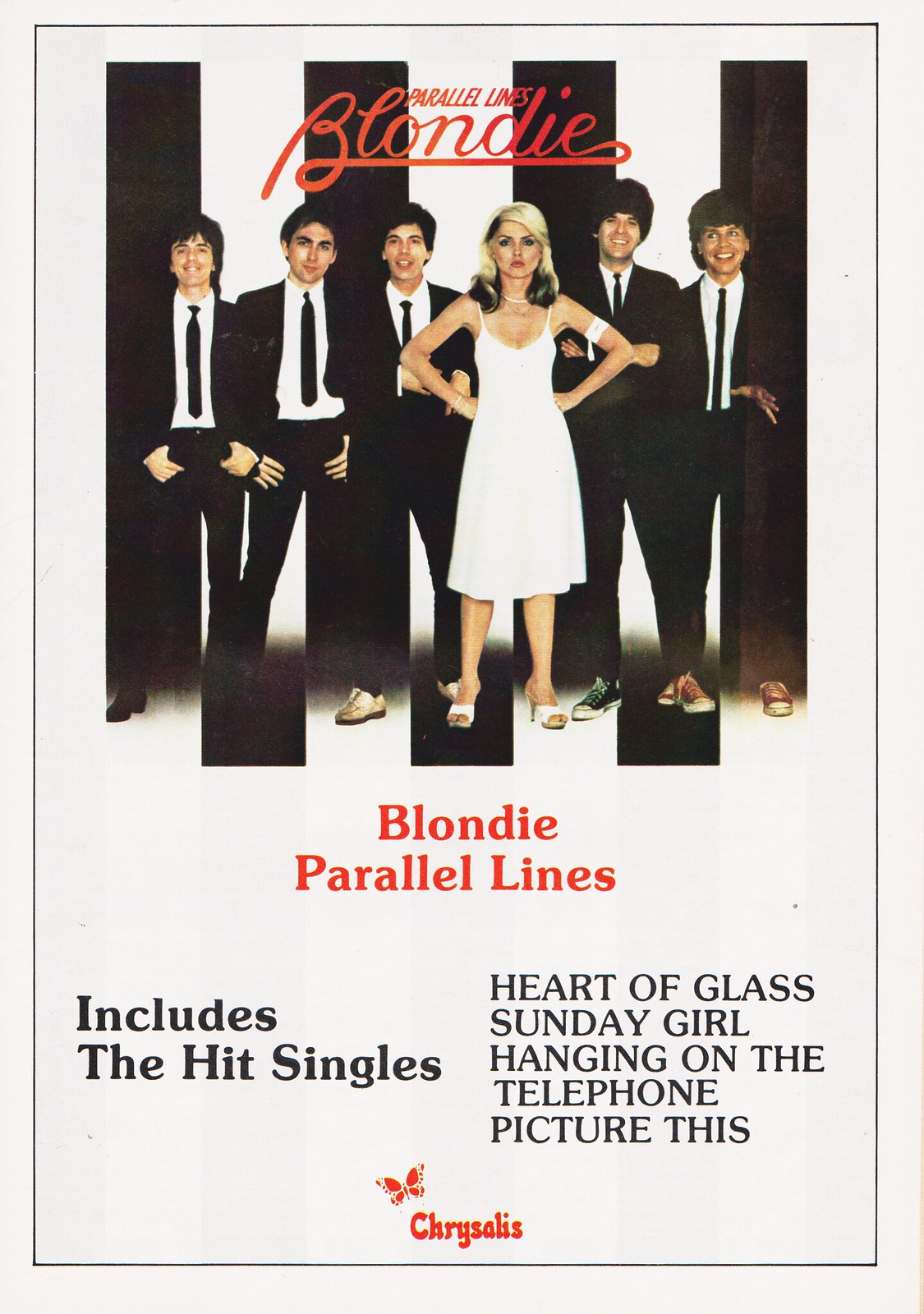This image is the album cover for Blondie's "Parallel Lines." It prominently features a color photograph of the band members standing side by side against a backdrop of alternating black and white vertical stripes. Debbie Harry, the lead vocalist, stands in the center, wearing a white dress with her hands on her hips. Her long blonde hair cascades down, and she is giving a stern look directly at the camera. Surrounding her are five male band members, all dressed uniformly in black suits, white shirts, black pants, and black ties, each sporting dark hair.

At the top of the photograph, "Parallel Lines" and "Blondie" are written in red text. Below the image, also in red text, it states, "Blondie, Parallel Lines," followed by a list of hit singles included in the album: "Heart of Glass," "Sunday Girl," "Hanging on the Telephone," and "Picture This." At the very bottom of the cover, there's a red logo of a butterfly next to the word "Chrysalis," the name of the record label. The composition and design elements of the cover, including the alternating stripe pattern, underscore the album's title, "Parallel Lines."